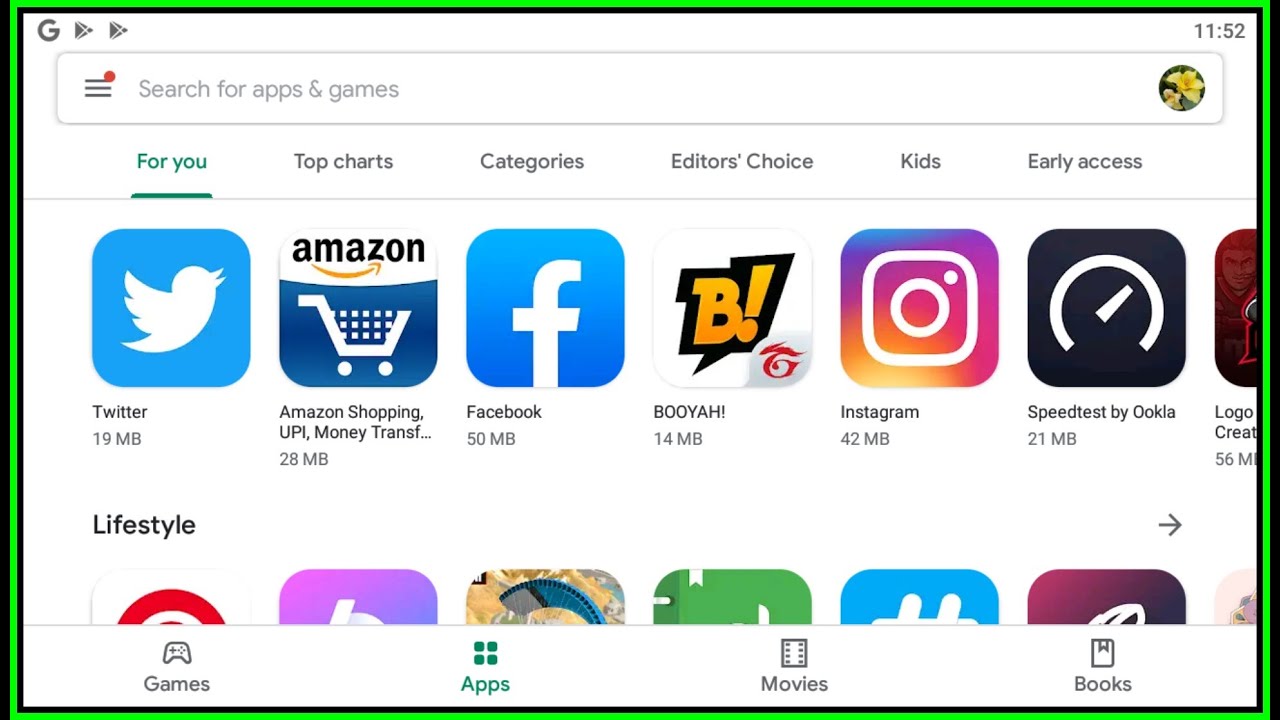The image is a screenshot of an application directory interface, likely from an app store or library. At the top of the interface, there is a prominently displayed search bar with the placeholder text "Search for apps and games." Below the search bar, there's a navigation tab labeled "For You", which is highlighted in a greenish color for emphasis. 

Displayed on the screen are a series of app icons with their corresponding names: Twitter, Amazon, Facebook, Puya, Instagram, and Speedtest by Ookla. The list continues, but the last visible app is partially cut off, and additional apps are also truncated, making their names unreadable. 

At the bottom section of the screen, there are navigation tabs for different categories: Games, Apps, Movies, and Books, providing easy access to various types of content within the app store.